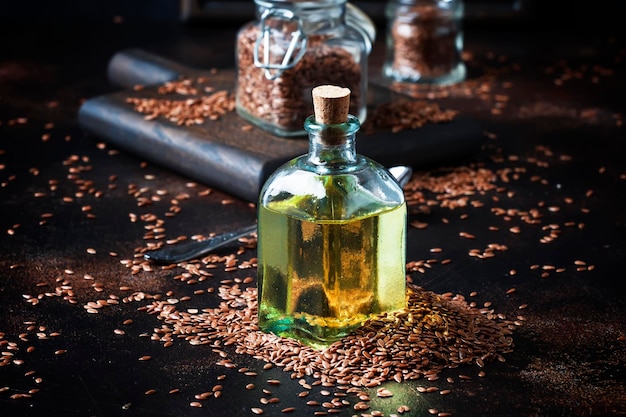The photograph features a central glass decanter filled with yellow, possibly sesame seed oil, sealed with a cork at the top. Surrounding the decanter on a black tabletop are scattered brown seeds, oval and long in shape, with some clustered in a pile next to the bottle. In the background, a dark oak cutting board hosts more seeds and a similar, smaller glass canister, this one sealed with a clasping lid. Another similar jar with a green tint is partially visible further behind, also containing seeds, creating a visually cohesive scene that highlights the different storage methods and the rich, earthy tones of the seeds and their containers.